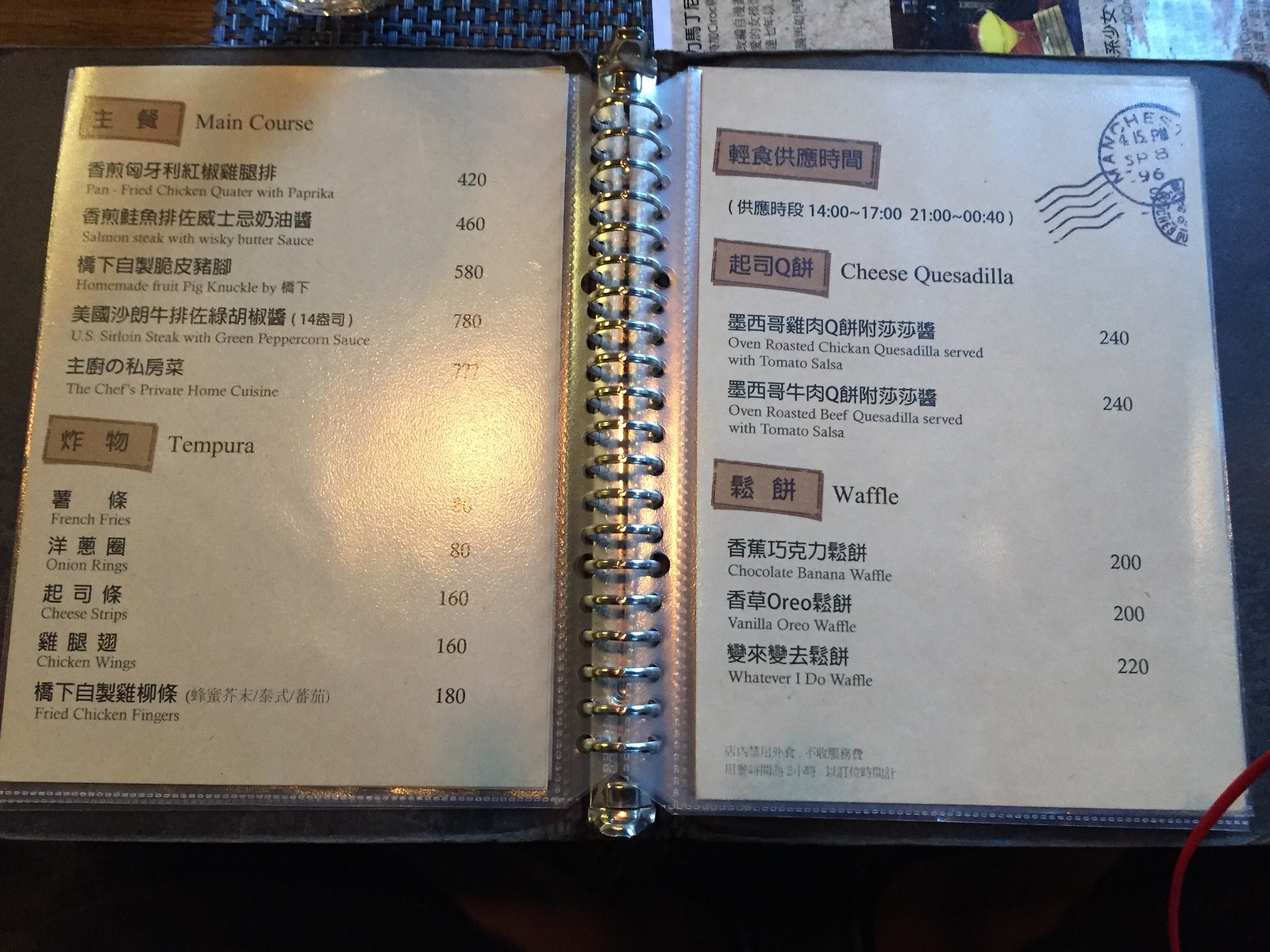The image captures an overhead view of a table setting, featuring a blue woven placemat laid neatly on a table. Partially seen is the bottom edge of a drink, suggesting a casual dining experience. Centered in the composition is a menu adorned with text primarily in Chinese or Japanese, interspersed with English phrases. The menu lists a variety of dishes with an intriguing range of prices. It highlights main courses such as pan-fried chicken with paprika priced at $4.20, alongside Chef's private home cuisine, which intriguingly lacks a price listing. Surprisingly high prices include French fries at $26.00, onion rings at $80.00, cheese strips at $160.00, chicken wings at $160.00, and fried chicken fingers at $180.00. Cheese quesadillas do not have a listed price, while oven-roasted chicken and beef quesadillas served with tomato salsa are both modestly priced at $2.40. Dessert options feature a chocolate banana waffle and a vanilla Oreo waffle, each at $2.00, and a whimsically named "Whatever I Do" waffle for $2.20. The menu, with its mix of exorbitant and reasonable prices, suggests it might be outdated or serve as a unique artifact in this dining establishment.